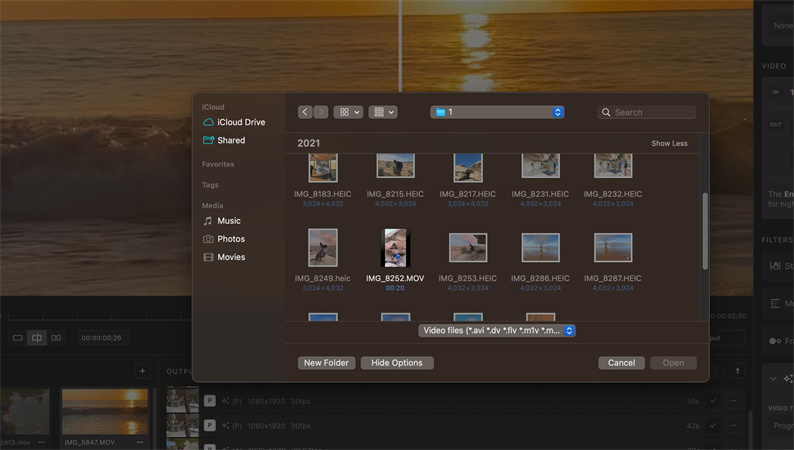This image is a detailed screenshot of an iCloud Drive interface on a computer, set against a predominantly brown background. The upper section of the background features an evocative image of a calm ocean with a peaceful wave rolling in. The scene is tranquil, with the sun setting in the distance, casting a shimmering reflection across the water towards the viewer.

In the forefront of the screenshot, a detailed brown rectangular pane occupies the center to the right side of the image, showcasing various icons, pictures, and text integral to the iCloud Drive interface. On the far left within this pane, a vertical sidebar lists the main sections: a light brown text label that reads "iCloud," followed by a blue cloud icon next to the label "iCloud Drive" in white text. Below that, another blue icon of a folder is alongside the "Shared" section in white text. Further down, there are brown text labels for "Favorites," "Tags," "Media," and specific categories such as "Music," "Photos," and "Movies."

To the right of this sidebar, the pane is organized into five horizontal rows displaying thumbnails of various media files like movies, clips, songs, and videos, providing a visual overview of the contents within the iCloud Drive.

At the top right corner of the pane, there is a convenient search bar, allowing users to locate specific files quickly. Towards the bottom of the pane, options for managing files are listed, including "New Folder," followed by "Hide Options." In the bottom right corner, functional buttons labeled "Cancel" and "Open" provide additional operational controls for file management within this interface.